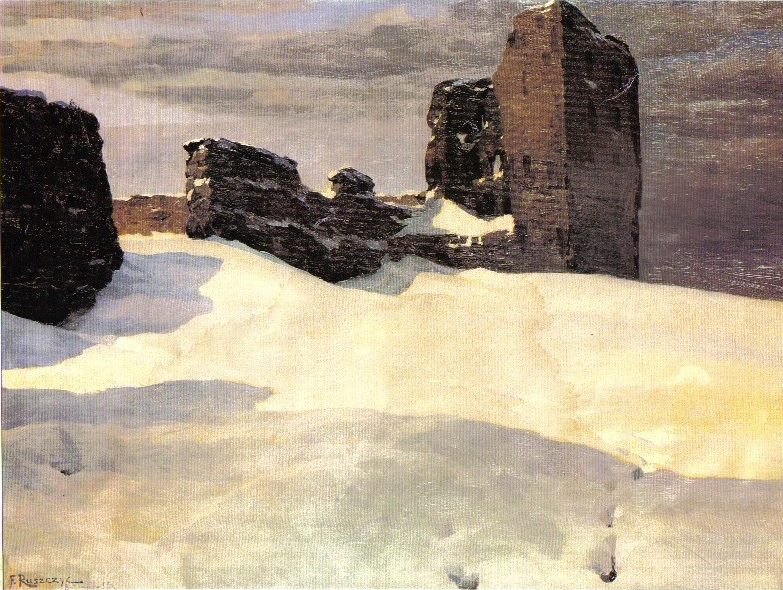This painting, likely an old piece given its visible canvas fibers and slight cracking, portrays a haunting, icy landscape dominated by jagged, dark rocks and snow-covered ruins atop a hill. The foreboding, cloudy sky thrusts ominous shadows across the scene, pierced by faint sunlight from the top left corner. The lower region features a blurry depiction of frozen water, textured with rough brush strokes hinting at underlying rocks. Prominent is a large, black, rhombus-shaped rock on the left, devoid of snow. Central in the composition is a partially-standing stone structure, its walls dusted with snow and comprised of a rectangular box and adjacent smaller shapes, including a pyramid-like form and a curved triangle. The backdrop remains stark and overcast, with a signature barely discernible at the bottom left, possibly reading "E or F R-U-S-E-C-R," adding to the painting’s mysterious allure.